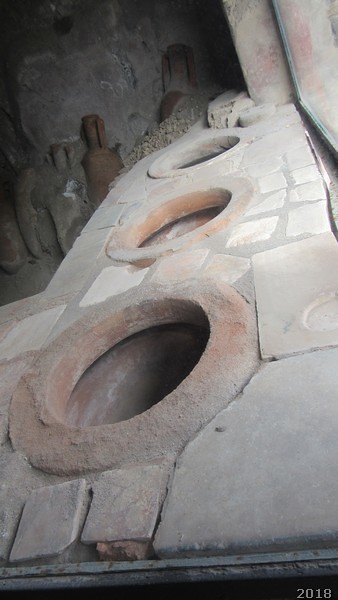The image depicts the interior of what appears to be an ancient or very old, dusty building, shown in a color photograph oriented in portrait mode. Dominating the foreground is a stone-paved basin or bench-like structure, comprised of square and rectangular stones, carefully arranged and set in place with a cement putty make the surface flat and level. Embedded within this bench are three large, circular ceramic holes aligned in a row, so deep that their bottoms are not visible. 

The backdrop features a dark stone wall, partially crumbled and covered in rubble. Leaning against this wall are a number of ceramic pots or vases, some of which are also crumbling. To the right of the scene, bits of glass suggest the presence of a window, albeit a partially shattered one. The entire setting is composed of terracotta-colored stones and pavers, contributing to the ancient and dusty ambiance. Additionally, the bottom right corner of the image features a white date inscription reading "2018." There are no people or animals present in this photograph.